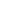In this black and white photograph, a young boy, who appears to be either of Asian or Native American descent with medium-length black hair, is captured in the midst of shooting a homemade slingshot. He is wearing a long sleeve button-down shirt with pockets on both sides, a white t-shirt beneath, and dark, likely black, pants held up by a belt. His clothing appears slightly dirty, consistent with an outdoor, rural setting. The boy, intensely focused, pulls back the black rubber strap of his Y-shaped wooden slingshot, aiming it with precision towards an unseen target. He stands amidst tall grass and various plants, with a simple wooden cabin, reminiscent of a structure from the 1940s or 1950s, seen in the background. The image, with its detailed depiction and thoughtful composition, evokes a sense of rustic simplicity and timeless childhood moments.